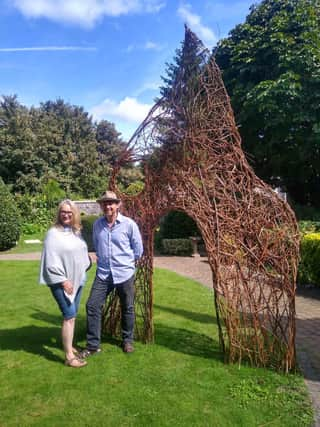A man and a woman are standing outdoors next to a large, artistic tree arch in a garden on a sunny day. The arch, made of twisted branches, is shaped like a doorway and stands about twice their height. The woman stands to the left, wearing white sandals, blue shorts, and a white top, with long blonde hair and glasses. The man, to the right, is dressed in a light blue shirt, black jeans, black boots, and a hat. They are positioned on green grass beside a walkway made of stone bricks. In the background, there are scattered clouds against a bright blue sky, a tree line, and a small fountain behind the arch. The scene resembles a pleasant backyard setting with various bushes and trees enhancing the serene atmosphere.